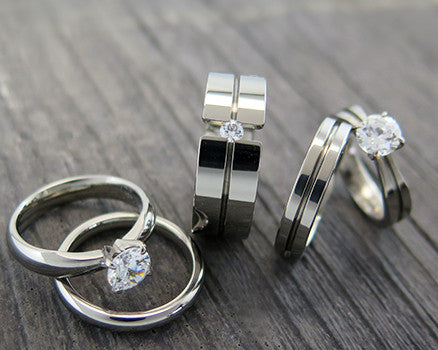This image is a color photograph in landscape orientation, depicting an arrangement of five silver rings on a dark brown, weathered wooden surface. The photograph emphasizes the intricate details and craftsmanship of each ring, captured in a representational, realistic style befitting product photography.

On the left side of the image, there is a set of two rings. The engagement ring, featuring a center stone with a four-prong setting, rests behind and slightly above the wedding band. Both rings lie flat on the wooden surface, showcasing their elegant design.

At the center of the photograph stands a wider, two-band configuration with a small silver or transparent stone in the middle. The bands interlock seamlessly, and the rings are positioned upright with the stone pointing upwards, drawing attention to their intricate interlocking design and the subtle diamond.

On the right side, another two-piece set is prominently displayed. The engagement ring, adorned with a solitary diamond, stands on its end, leaning slightly towards the accompanying wedding band. Both rings are positioned to highlight their complementary engravings and the sparkling gemstone.

The entire composition is illuminated with subtle light, accentuating the textures of the gray, weathered wooden backdrop and the gleaming silver bands. The photograph exudes a sense of timeless elegance and refined craftsmanship.